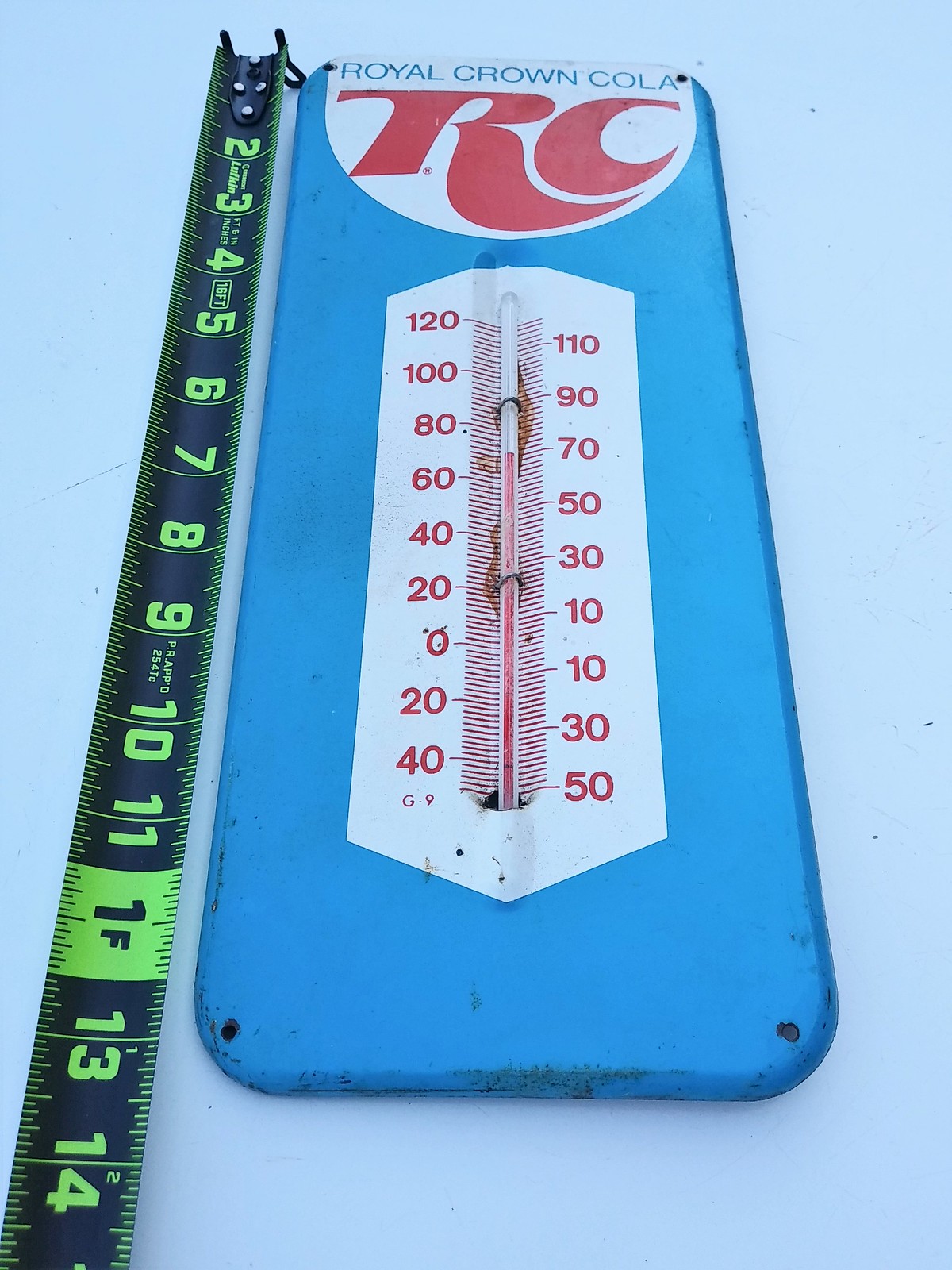The photograph features a rectangular object prominently displaying the title "Royal Crown Cola" and the initials "RC" in bold red letters. Inside this rectangular object is a smaller item, a thermometer, clearly showing its gradients and containing liquid mercury in the center. Adjacent to the thermometer, a black ruler marked with green numbers and reading lines measures the length of the rectangular object. All these items rest on a very light blue surface adorned with black spots or markings. The detailed measurement and positioning provide a clear view of both the thermometer and the ruler alongside the "Royal Crown Cola" branding.